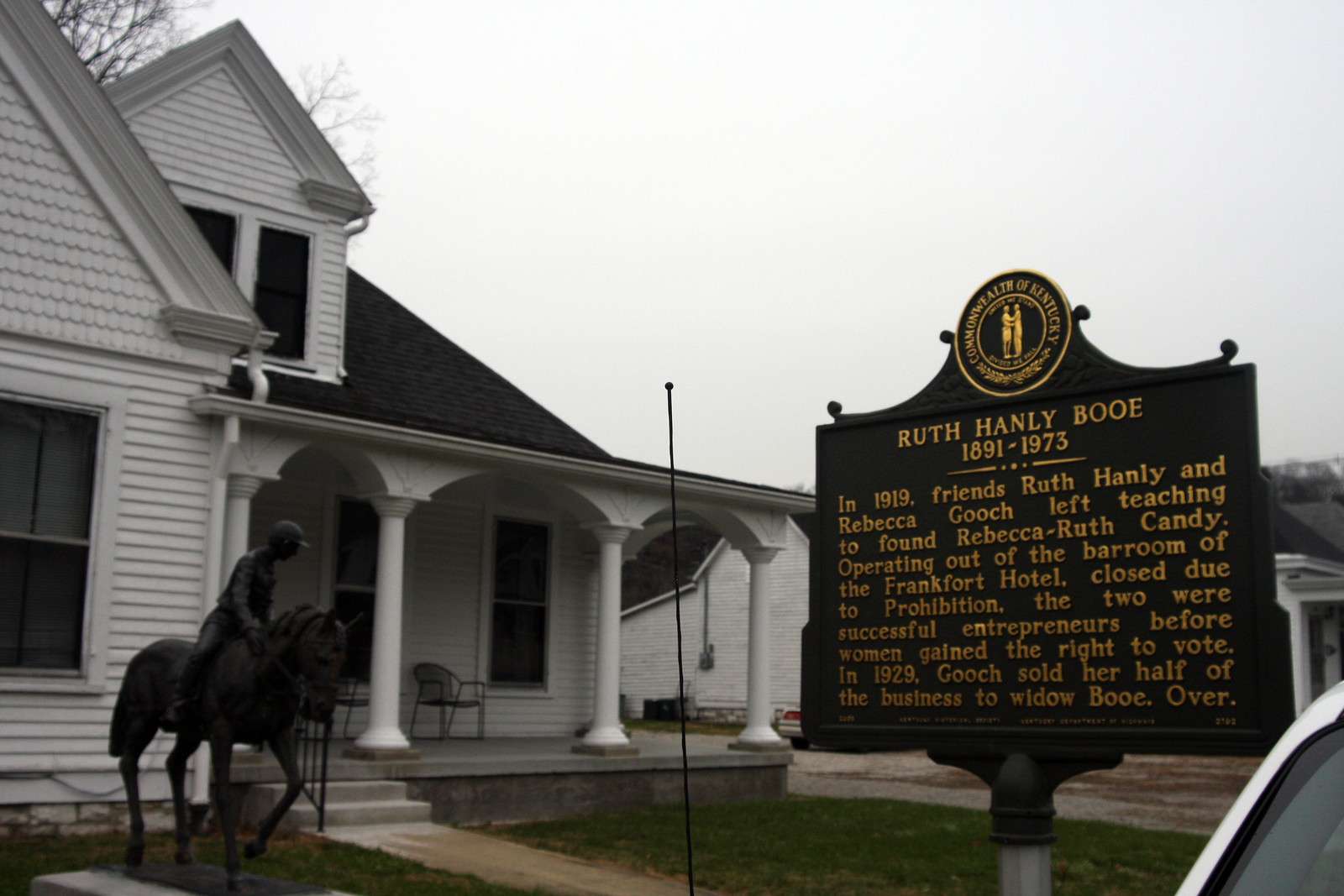The image depicts an outdoor scene featuring an old, white house with a black roof under an overcast, gray sky. The house appears quite large and has a patio area with visible steps and two chairs. In front of the house, positioned to the left, stands a black statue of a boy on a horse, adding a historical ambiance to the setting. To the right in the foreground is a black plaque with gold writing, including a circular symbol at the top that shows two gold figures embracing and the text "Commonwealth of Kentucky."

The plaque bears an inscription that reads: "Ruth Hanley Bowie, 1891-1973. In 1919, friends Ruth Hanley and Rebecca Gooch left teaching to found Rebecca Ruth Candy. Operating out of the ballroom of the Frankfurt Hotel, closed due to prohibition, the two were successful entrepreneurs before women gained the right to vote. In 1929, Gooch sold her half of the business to widow Bowie."

Behind the house, there is part of a tree without leaves, hinting at fall or early spring, yet green grass still covers the ground. A car with windows and an antenna is barely visible on the edge of the image. This detailed photograph captures not only the physical elements of its subject but also the historical significance associated with the house and its former inhabitants.